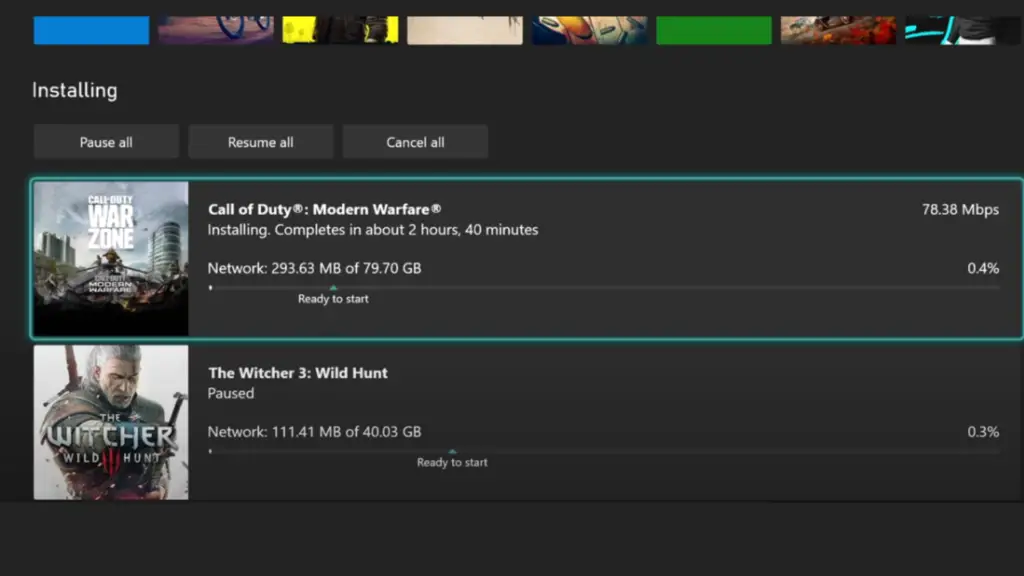This image depicts a screenshot of a gaming installation console interface, though the platform (PC, PlayStation, or Xbox) is not specified. At the top of the screen, there are several thin rectangles, including a blue one resembling a bicycle and others with abstract shapes that suggest a standing person, among other figures. Below these rectangles, there’s a green box which may represent different game titles. An installing icon is prominently displayed with three command buttons beneath it: “Pause All,” “Resume All,” and “Cancel All.”

To the left, there are thumbnails for individual games. The current selection is “Call of Duty Modern Warfare,” highlighted by a glowing blue outline. The screen reads, "Call of Duty Modern Warfare installing," with an estimated completion time of approximately 2 hours and 40 minutes. The download speed is indicated as 78.38 MB/s, and 293.63 MB of the required 79.70 GB have been downloaded so far. There is a progress bar showing that the game is "Ready to start" only a tiny portion of the way through the installation.

Below this, another game, “The Witcher 3: Wild Hunt,” is listed but paused. It shows 111.41 MB of the necessary 40.03 GB downloaded, with its "Ready to start" progress bar about a third of the way complete. All information is set against a background of various shades of grey.